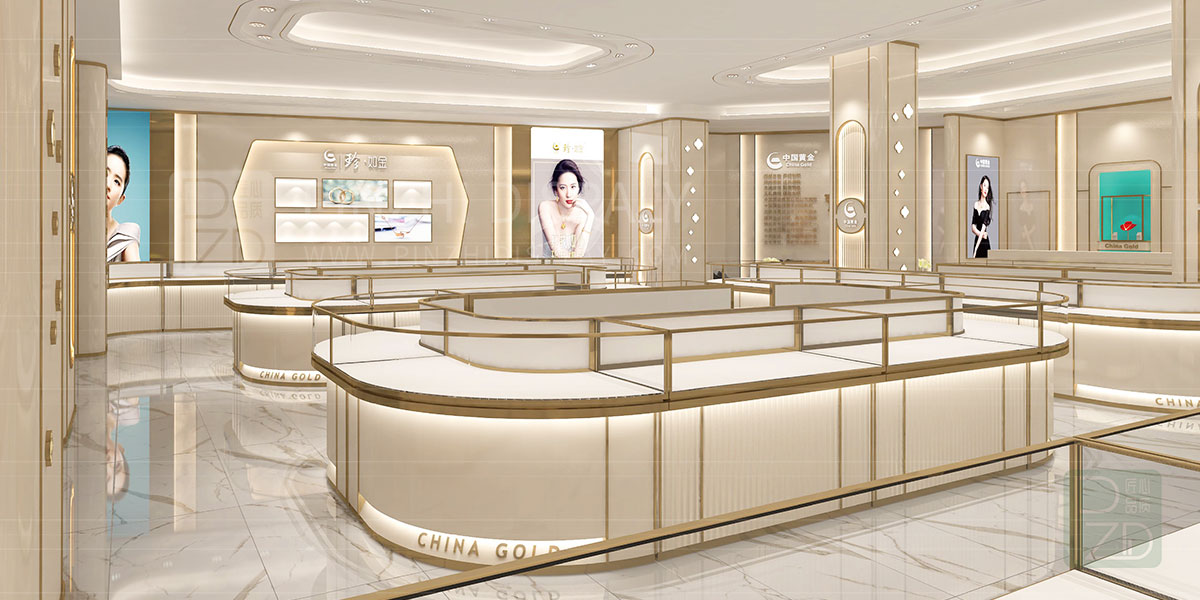This photograph captures a wide-angle view of an elegantly designed and meticulously illuminated jewelry store named "China Gold." The store's interior exudes opulence with its white marble floors accented by gold streaks and the matching white display cases adorned with gold trim. The display counters, which are topped with clear glass vitrines that remain pristinely empty, hint at the store's readiness for a grand opening. Intricately framed wall advertisements feature three striking images of Chinese women modeling jewelry, adding a stylistic flair to the space. These images are interspersed with Chinese lettering, possibly indicating the store's name or brand signature. The room's luxurious atmosphere is further enhanced by golden-hued pillars accented with gold trim, softly illuminated by strategic lighting that complements the overall aesthetic.